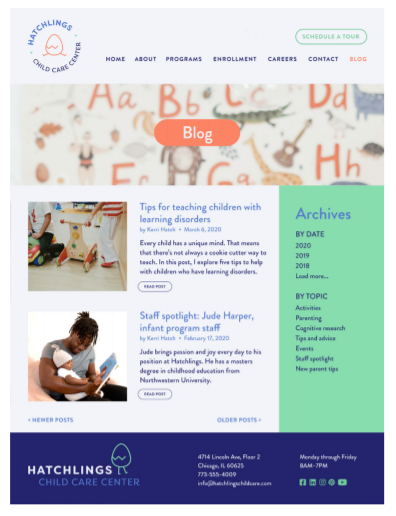The image is a screenshot from the website of a childcare facility named "Hatchlings Childcare Center." At the very top of the image, there is a logo depicting a small egg with a crack in it, encircled by the text "Hatchlings Childcare Center." The website's navigation bar includes links to various sections: Home, About, Programs, Enrollment, Careers, Contact, and Blog. There is also a button labeled "Schedule a Tour." The main section of the image appears to focus on the blog page, as indicated by the visible content.

This section features two blog posts, each accompanied by related images of children or babies. The first post is titled "Tips for Teaching Children with Learning Disorders," while the second highlights a staff member in "Staff Spotlight: Jude Harper, Infant Program Staff," with an image likely showcasing Jude Harper. On the right-hand side of the page, there is an archive section allowing users to browse posts by date, specifically from the years 2020, 2019, and 2018. Another section organizes posts by relevant topics, such as children, parenting, and activities.